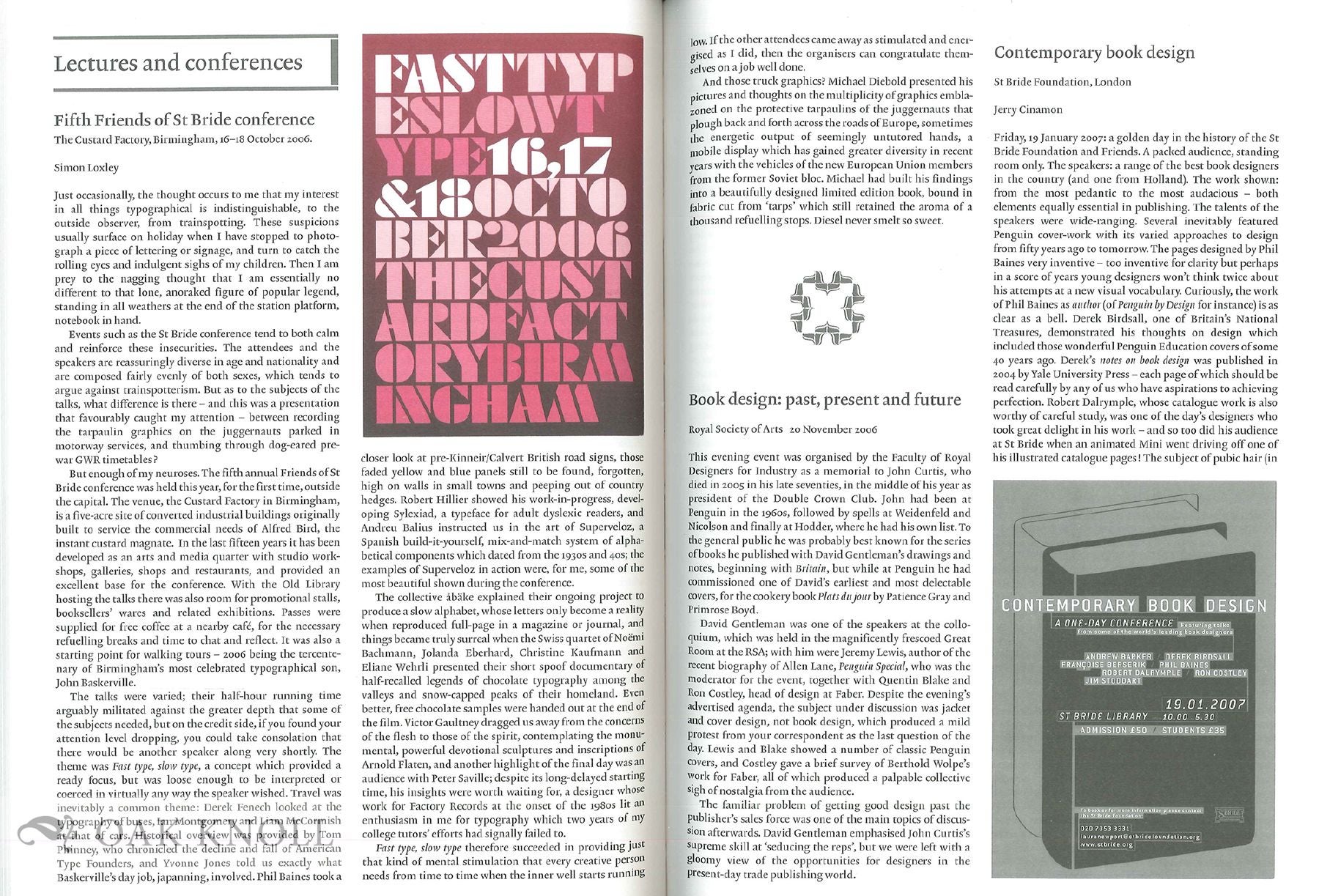This image shows an open book, revealing both the left and right pages, featuring the inside contents of a magazine or possibly a book. The pages are white with very small black text. At the top left of the left page, there is a heading in larger text, "Lectures and Conferences", followed by "Fifth Friends of St. Bride Conference", detailing the location as "the Custard Factory, Birmingham" and the dates "16th to 18th of October, 2006". Below is an article that reflects on typographical interests, mentioning the poster for the conference with distinctive stencil-style letters blending into each other, accompanied by an anecdote about the author's passion for typography.

The right page also includes text discussing various topics such as book design. There is a reference to another event, "Book Design: Past, Present, and Future" at the Royal Society of Arts on "20th November 2006". Further down, a small icon represents "Contemporary Book Design: A One-Day Conference", scheduled for "1901-2007".

The left side of the left page features another section with the title "Fast Type, Slow Type", reiterated with information similar to the introductory section, and functioning as a visual element akin to a conference poster. Additionally, to separate the sections on the right page, a small decorative graphic is included. The overall spread appears dense with informative text about various conferences and events centered around typography and book design.